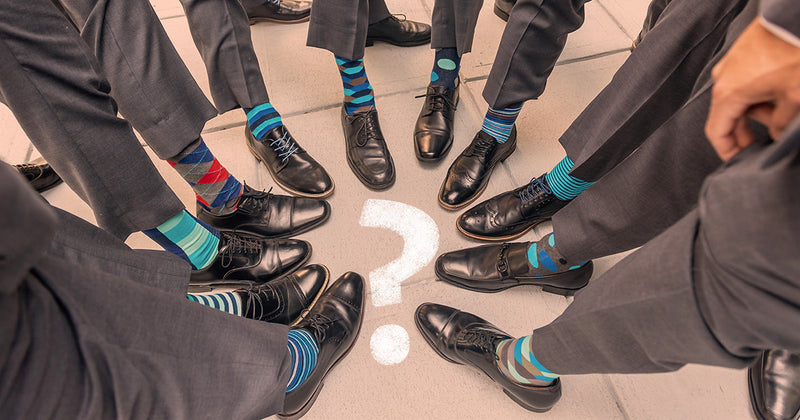This animated image depicts the lower legs of approximately 9 to 11 individuals, all standing in a circle on a light pink tile floor. The focal point of the image is a large white question mark at the center of their circle. Each person is wearing black suede dress shoes, with most featuring black shoelaces, though two pairs have unique light blue and dark blue laces. The individuals are all dressed in gray dress pants and their socks, predominantly featuring shades of blue, exhibit a variety of patterns including stripes, argyle, and polka dots. The clean, minimalistic arrangement and cohesive attire draw attention to the central question mark, creating a thoughtful and visually engaging composition.